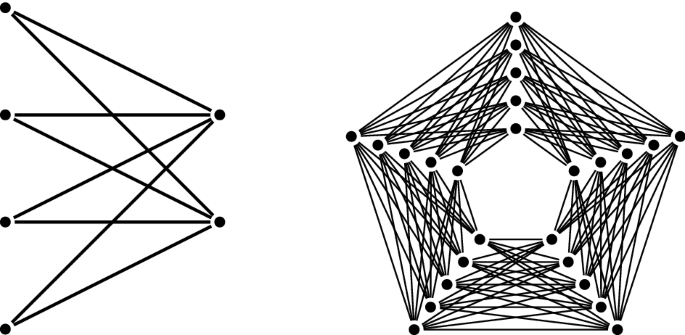The image features two geometric drawings showcasing symmetry, rendered in black on a white background without any borders or text. The left side displays a trapezoidal configuration composed of six dots. Four dots are aligned vertically on the extreme left, with two additional dots positioned horizontally to the right. Black lines connect these dots, forming a complex pattern of overlapping triangles, resembling a connect-the-dots puzzle. The right side presents a pentagonal figure made up of 25 dots arranged in a star-like pattern. The dots outline a pentagon, with each dot connected by black lines to others at equal intervals, creating a dense network of overlapping triangles while leaving the center of the pentagon as empty white space. Both images highlight intricate patterns formed through strategic dot and line placement, evoking a crocheted string appearance.